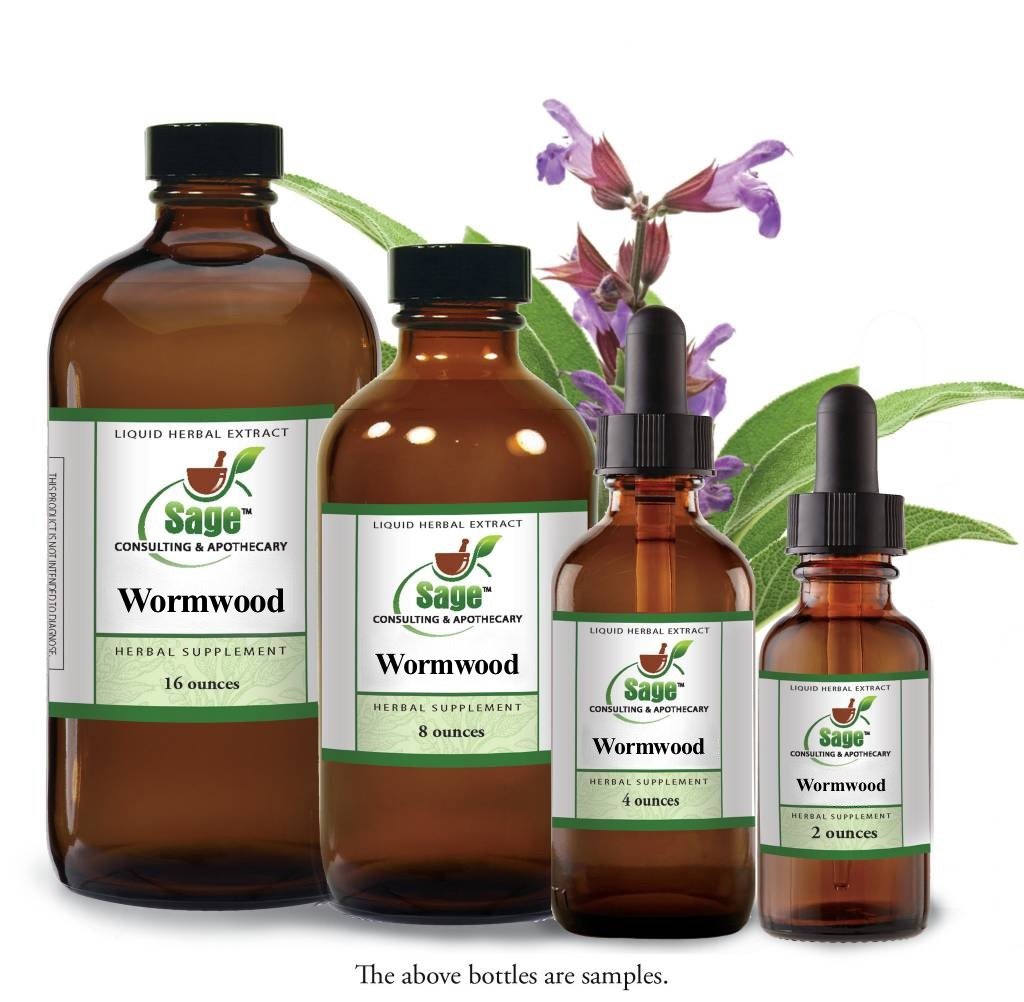The photograph features four amber-colored medicinal bottles designed for storing light-sensitive substances like essential oils. The largest bottle on the left, with a black screw-on cap, holds 16 ounces and is labeled "Liquid Herbal Extract" from Sage Consulting and Apothecary. This wormwood herbal supplement is clearly indicated on the label, which features a mortar and pestle logo. Beside it stands a sequentially smaller 8-ounce bottle with an identical screw-on cap and label. The next bottle, holding 4 ounces, switches to an eyedropper-style top for precision dispensing, as does the smallest 2-ounce bottle. All bottles share the same white label branding: "Sage Consulting and Apothecary - Wormwood Herbal Supplement." Behind this array, a sprig of sage or salvia, signified by its fuzzy long leaves and purple tubular blooms, suggests the origins of the product. Below the bottles, a caption notes, "the above bottles are samples."